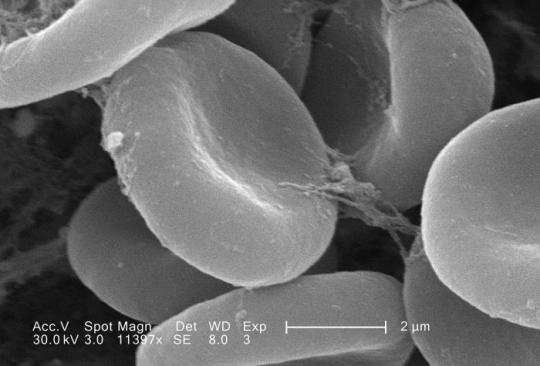This intriguing black-and-white microscope image, likely captured using a Transmission Electron Microscope (TEM) with a high 11,397X magnification, showcases cellular structures. The focus is on numerous red blood cells, identifiable by their distinctive concave, circular shape. The 3D imaging allows a clear visualization of the cells' crescent-shaped indentations. A scale bar at the bottom of the image indicates dimensions of two micrometers, alongside additional annotations including exposure (Exp3), working distance (WD 8.0), detector type (SE), and accelerating voltage (ACC.V 30.0 KV). This detailed microscopic view lacks the characteristic red color of blood cells, as it is presented in varying shades of black and gray.